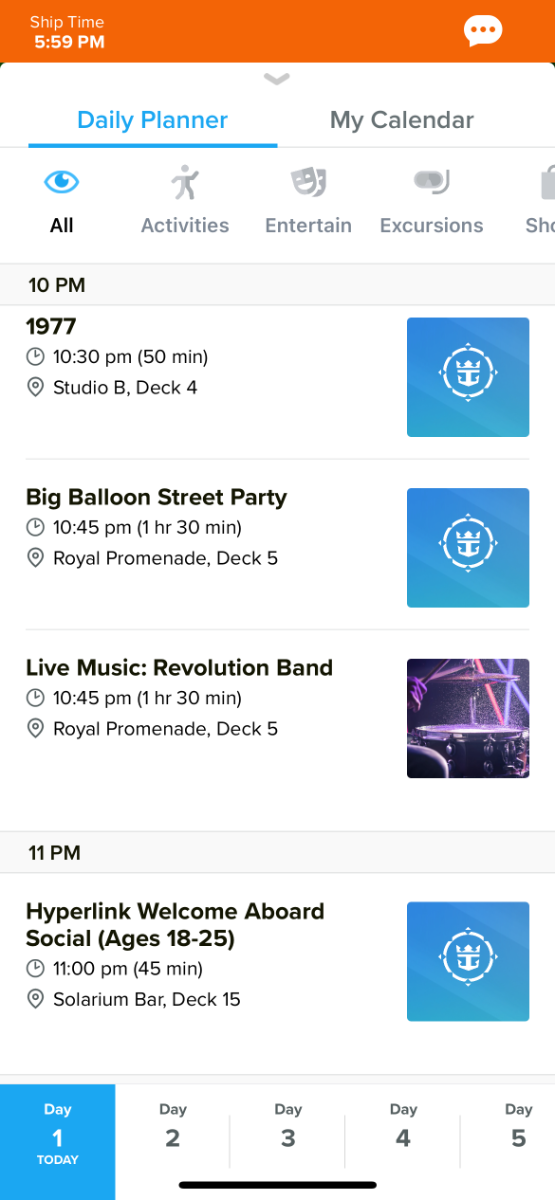**Detailed Caption:**

This image showcases a daily planning app for a smartphone, displaying a list of scheduled events with their corresponding times and locations. At the top of the screen, there is an orange bar featuring white text on the left side that reads "Ship Time," with "5:59 PM" displayed directly below it. Adjacent to this, a white conversation bubble containing three orange dots is visible, indicating potential new messages or notifications.

Below the bar, two options are available: "Daily Planner," which is highlighted in blue, and "My Calendar," which is grayed out and not selected. These options are part of a navigation menu which includes five icons labeled "All," "Activities," "Entertainment," "Excursions," and "Shopping." The icons are paired with corresponding text and symbols, although the "Shopping" section is partially cut off.

The event list begins with a 10:00 PM entry titled "1977," noted to last for 50 minutes until 10:30 PM. The location is specified as "Studio B, Deck 4," and a blue box with a white shield icon is present to the right. This is followed by the "Big Balloon Street Party," scheduled for 10:45 PM with a duration of one hour and 30 minutes at the "Royal Promenade, Deck 5." It also features the same blue shield icon.

Continuing down the list, "Live Music: Revolutionary Band" is mentioned with a start time of 10:45 PM, lasting for one hour and 30 minutes at the "Royal Promenade, Deck 5." This entry includes a small, colorful image suggestive of a stage. The final event listed is the "Welcome Aboard Social (Ages 18-25)" at 11:00 PM, lasting 45 minutes at the "Solarium Bar, Deck 15." The time and event name are hyperlinked, presumably for additional details.

At the bottom of the app interface, there are five labeled boxes representing different days: "Day 1 (Today), Day 2, Day 3, Day 4, and Day 5," allowing users to navigate through the schedule of events for the entire cruise trip.